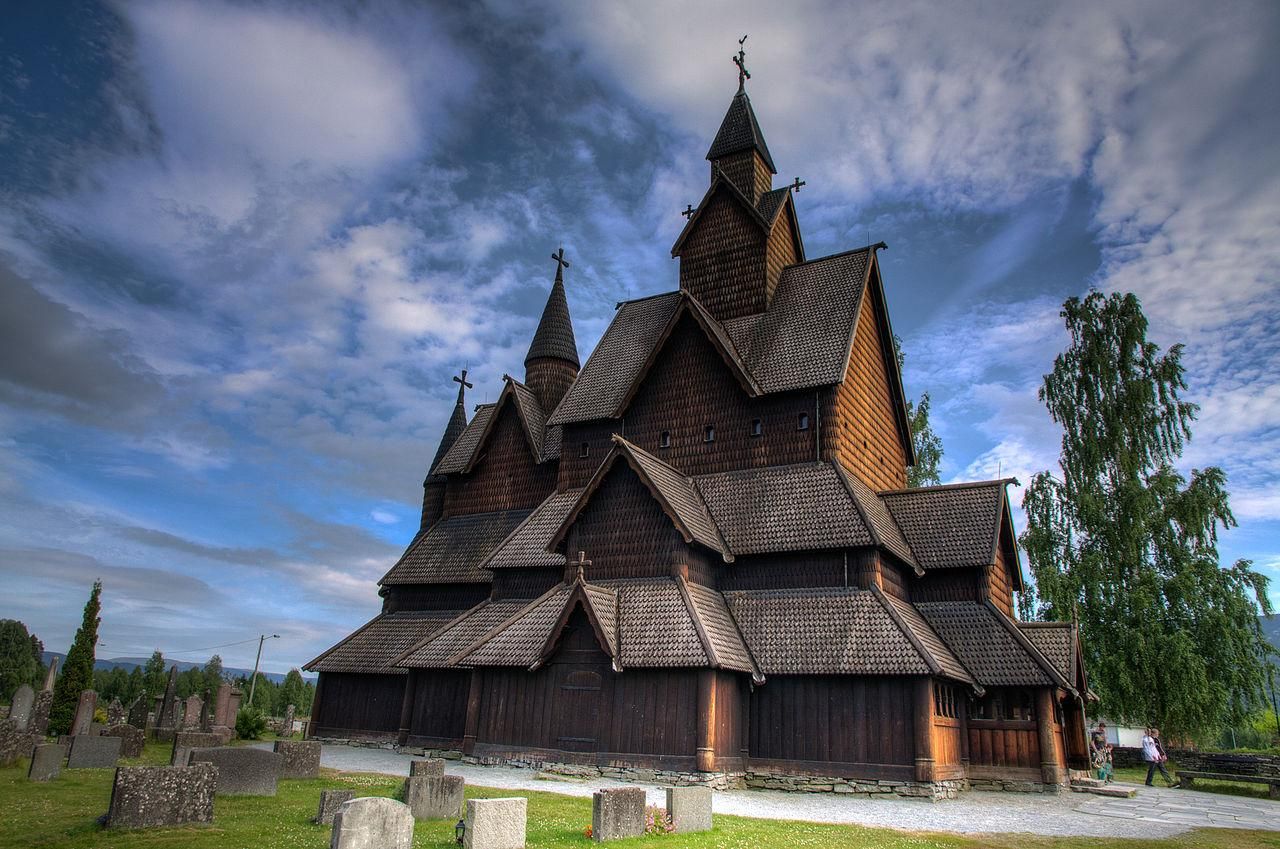The photograph depicts an old, rustic church under a blue, partly cloudy sky. The church is a striking multi-tiered structure in various shades of brown, made primarily of wood. It has five distinct layers, each progressively narrower as they ascend. The bottom layer of the church is very wide with steeply slanted roofs. The second story, also triangular with steep roofs, is narrower than the first. At the top, the church features three house-sized sections with extremely narrow roofs. The fourth layer has a single building with a triangular roof, and the fifth, uppermost layer is a tower crowned with a cross.

The foreground of the image shows a graveyard with rows of old stone gravestones arranged among lush green grass. Specifically, the left portion of the image includes several rows of gravestones: four in one row, three in another, and then two or three gravestones per row in the following rows. On the right side of the image a tall green tree is visible, and small figures of people can be seen in the background. Overall, the photograph captures the serene and slightly eerie atmosphere of an old church surrounded by history.